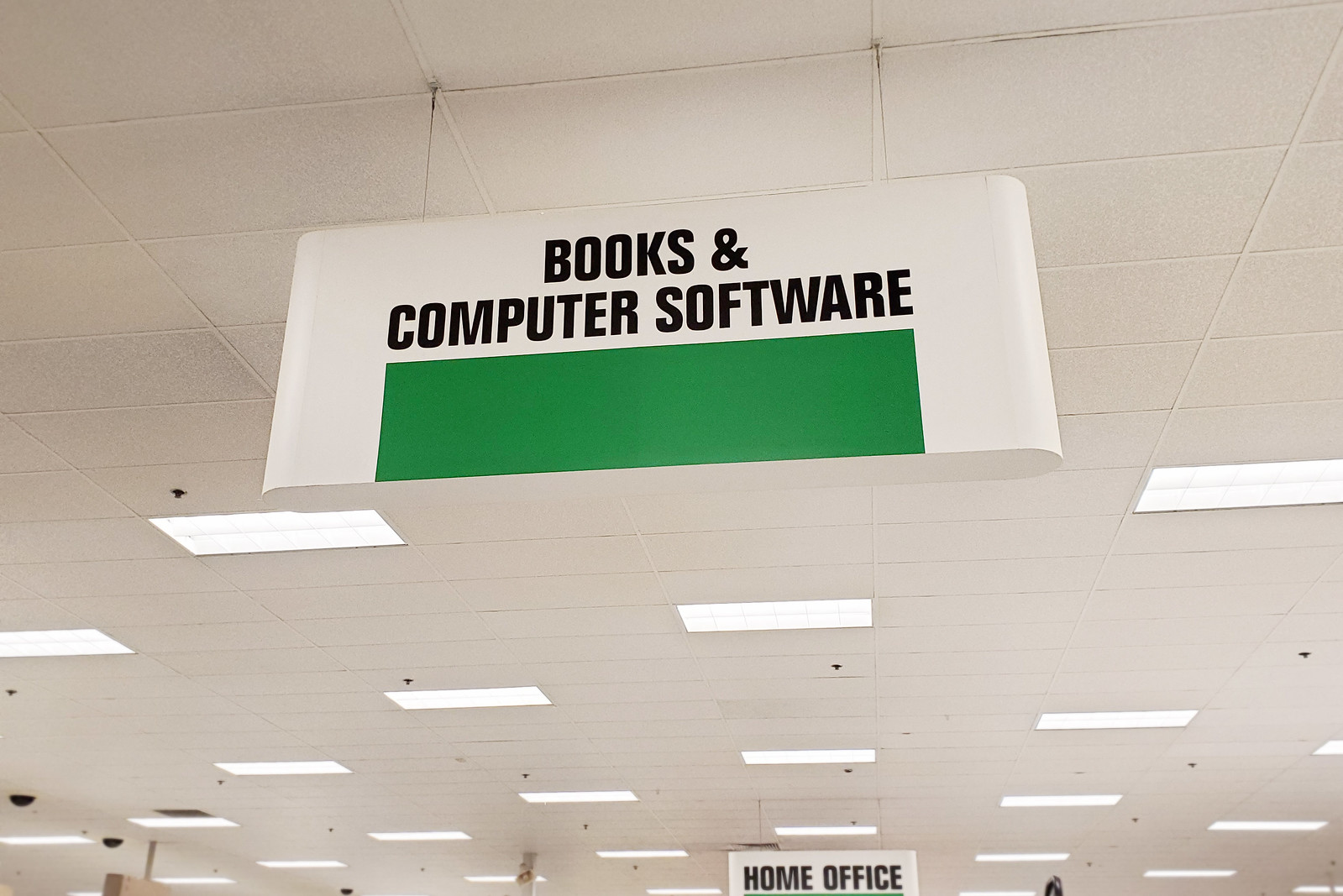This photo captures the ceiling of a retail store, showcasing a grid-like pattern composed of large, rectangular, white fiberboard tiles. Interspersed among the tiles are rectangular fluorescent light fixtures, providing even illumination throughout the space. The focal point of the image is a prominently displayed, white rectangular sign with rounded edges, presumably made of plastic. The sign, printed in bold black text, reads "Books and Computer Software," and features a green rectangular bar beneath the text for a touch of color contrast. In the background, partially visible, is another sign that reads "Home Office."